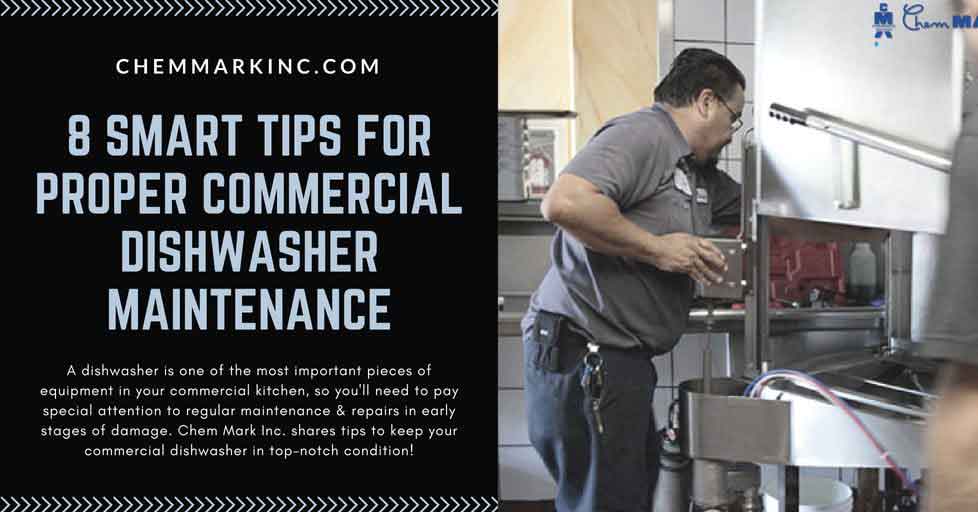The image is a modern advertisement for Chemmark Inc., featuring their website, chemmarking.com. On the right half of the rectangular ad, a heavyset gentleman service technician is deeply engrossed in repairing an industrial dishwasher. He is attired in work pants with keys attached to his belt loop and a tucked-in work shirt displaying his name tag. The left half of the ad contains textual information on a black background. The company's website is prominently displayed in white at the top, followed by the title "Eight Smart Tips for Proper Commercial Dishwasher Maintenance" in light blue. Beneath this title, a paragraph in light blue text emphasizes the importance of regular maintenance and early repairs for commercial dishwashers, describing them as crucial kitchen equipment. It further mentions that Chemmark Inc. provides tips to keep your commercial dishwasher in top-notch condition. The logo of the company is situated at the top right corner, resembling a stick figure with an exaggerated M-shaped torso, appearing to hold the company's name.